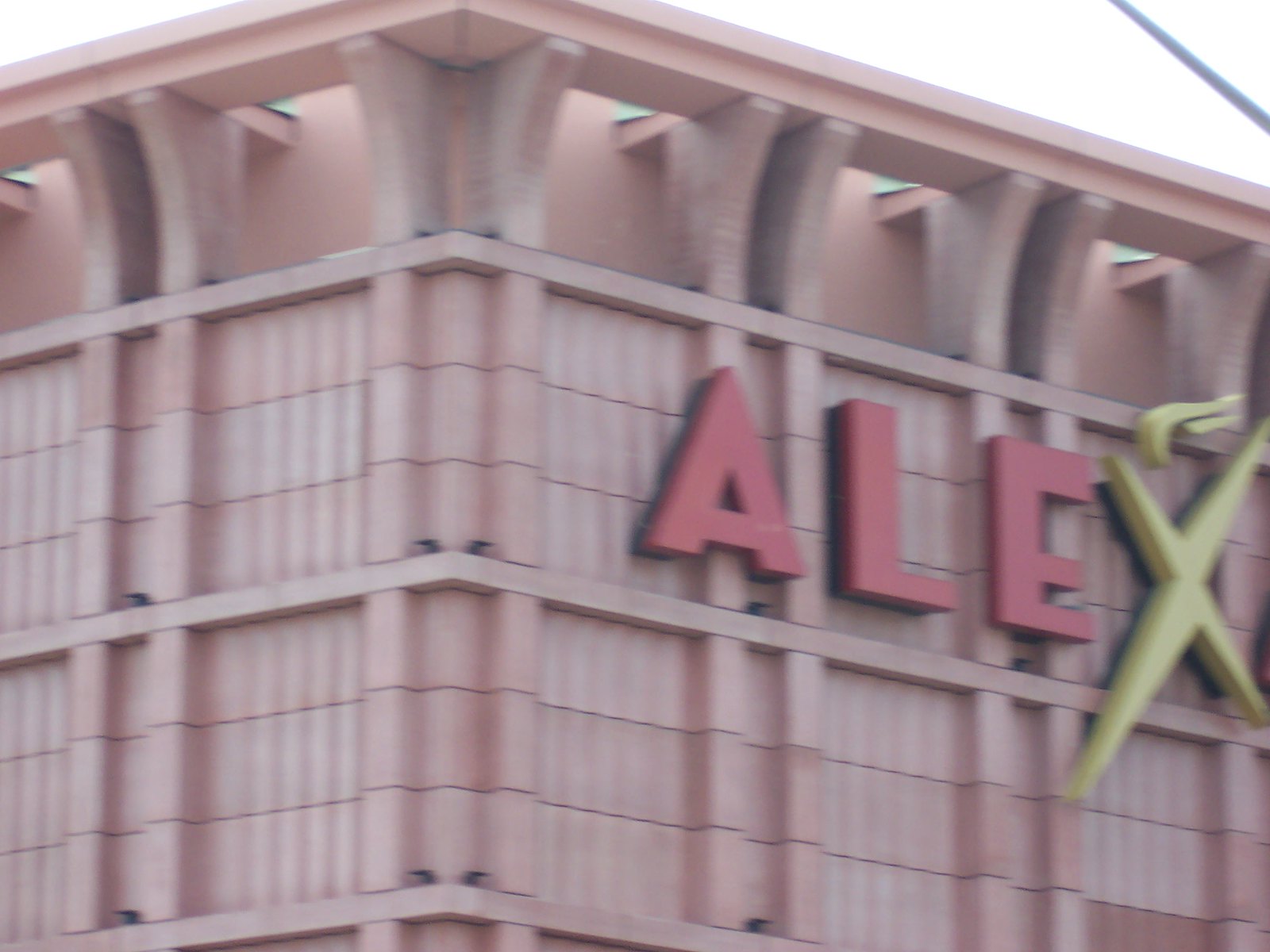The image captures the exterior of a tall, rectangular building with a light pinkish-salmon hue, possibly made of concrete shaped like bricks. The structure features distinct columns along its corners and sides, with each story marked by square sections that resemble blocks, making it appear stone-like. Prominently displayed on the building's right-hand side is the name "Alex." The letters "A-L-E" are in bold red, while the "X" stands out in a bright yellowish-green with an accompanying wind-like symbol in the same yellow hue, giving it a dynamic appearance. Above the building, a gray sky looms, and bright light peeks through the top left and top right of the image. Despite the photo being slightly out of focus, the building's architectural details and unique signage are clearly visible.